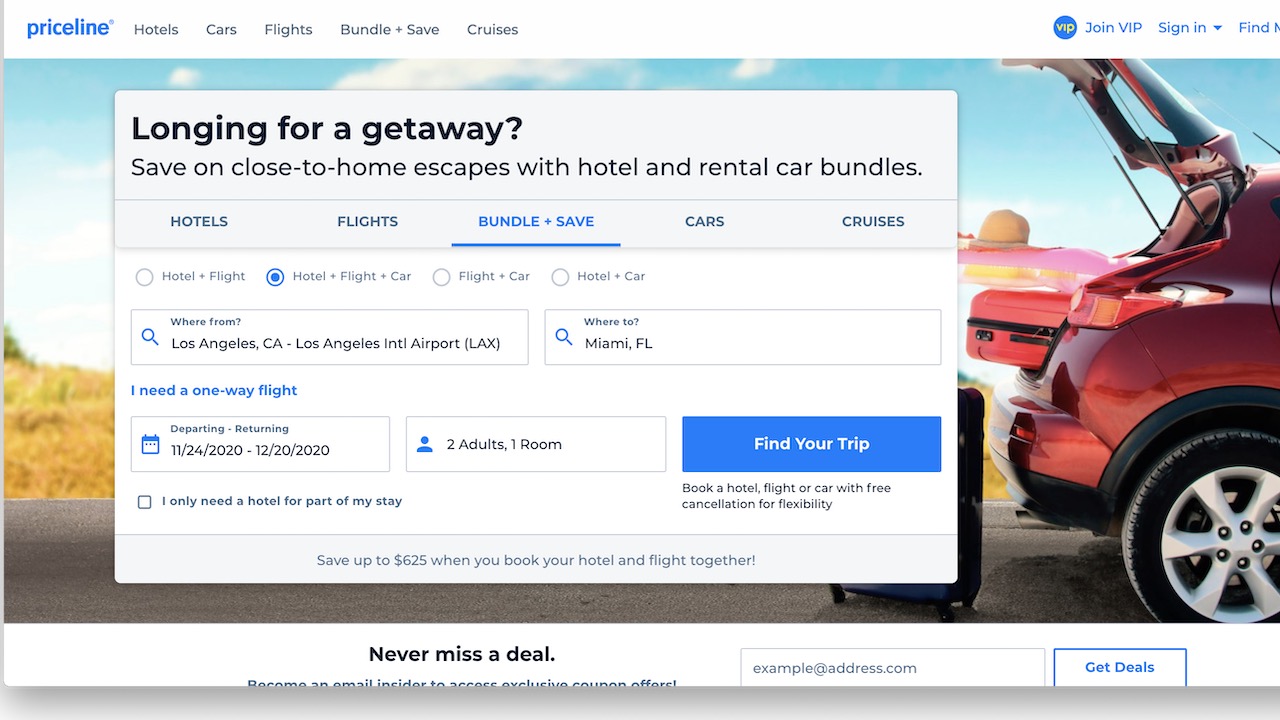Screenshot of a travel booking website featuring a prominent "Priceline" header in blue font with all lowercase letters. The navigation tabs include options for "hotels," "cars," "flights," "bundle & save," and "cruises." On the far right, there's a section for "VIP," "join VIP," and "sign in," followed by a "find" button that is partially cut off.

The background image shows a person standing by a road, next to a red SUV with its rear door wide open. They appear to be loading or unloading suitcases into the vehicle. 

A large overlaying rectangle in the center of the image displays a promotional message: "Longing for a getaway? Save on close-to-home escapes with hotel and rental car bundles." Below this message are tabs labeled "hotels," "flights," and "bundle and save," with the last one underlined in blue, indicating the selected option. Additionally, there are fields for selecting a one-way flight, with options for specifying the departure and arrival locations.